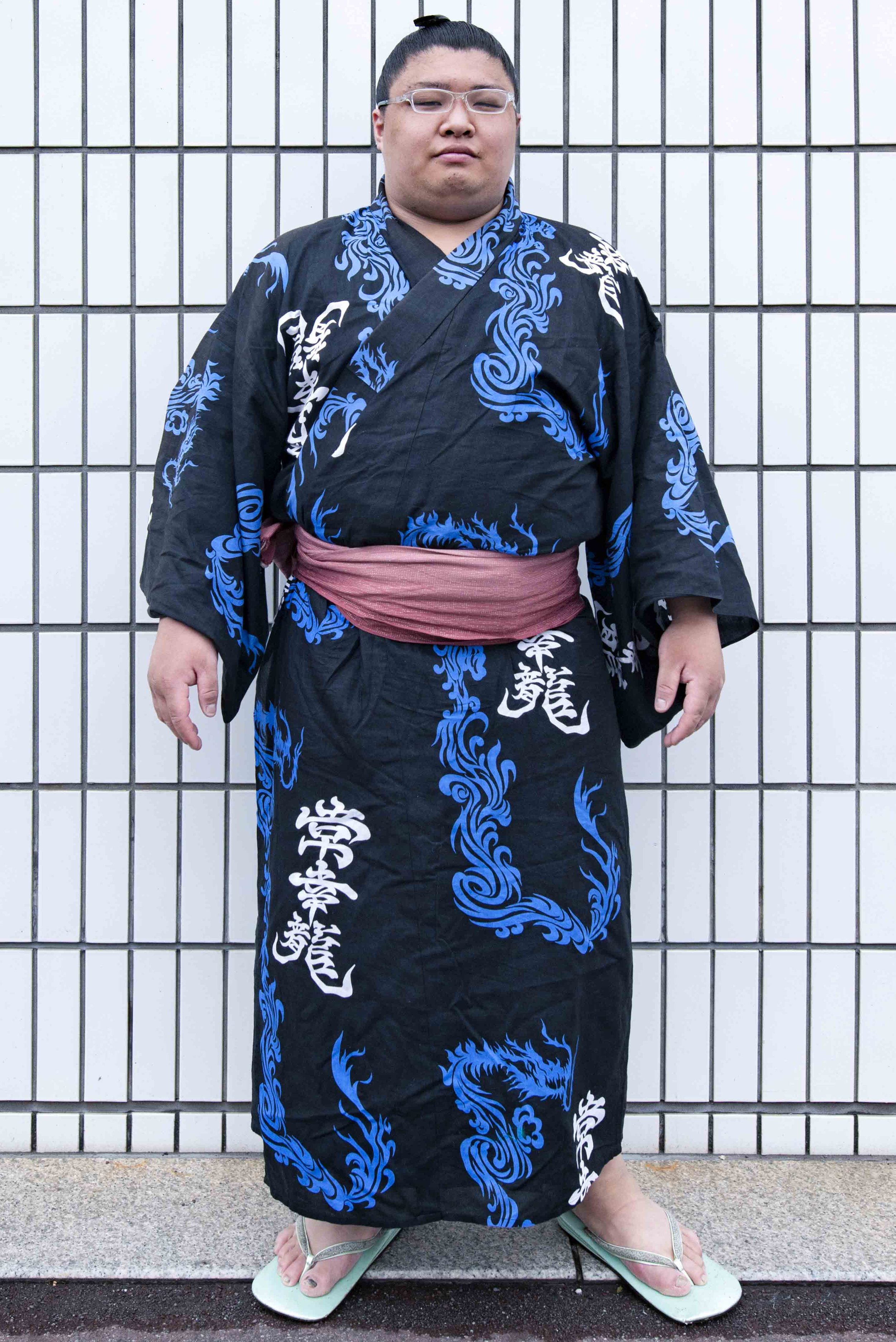The image is a color photograph in portrait orientation, capturing an Asian individual, possibly a sumo wrestler, who appears to be around 30-35 years old. The person stands confidently, facing the viewer, adorned in a black wraparound kimono. The kimono features intricate white and blue dragon patterns and additional white text in Asian script. A red sash, tied at the waist, adds a pop of color to the ensemble. The individual's dark hair is styled in a bun, and they wear distinctive white wire-rimmed glasses. Their feet are clad in aqua-colored flip-flops, complementing the kimono that extends down to their ankles. Positioned against a traditional shoji screen with a black and white grid pattern, they stand on a pebbled granite surface. The scene exudes an atmosphere of photographic realism, capturing the subject in a poised and elegant fashion.